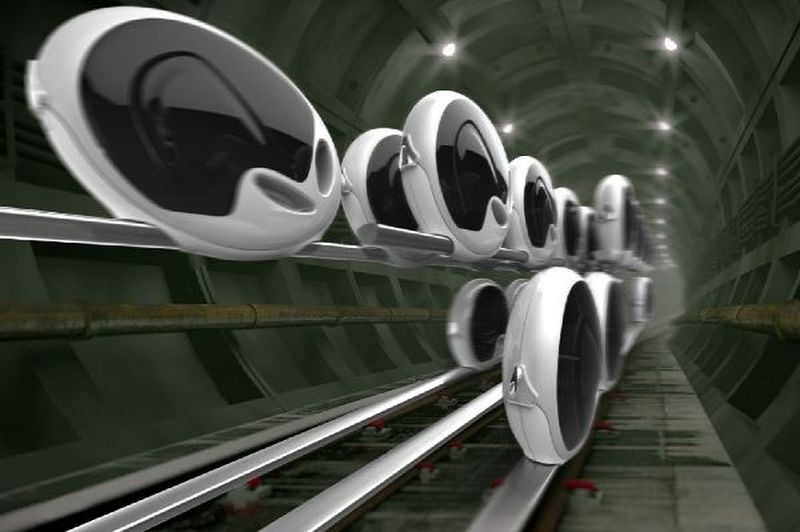In this detailed black and white photographic image, we view a futuristic indoor scene from the vantage point of someone standing at the beginning of a tunnel. The tunnel, possibly a depiction of a mass transit or subway system, showcases polished steel rails extending into the distance under a string of lights, culminating in a gray opening at the tunnel's end. The rails support a series of shiny silver wheels with black inlays, arranged in two staggered rows – approximately 12 in total, with three or five on the bottom rail and the rest on the upper rail. To the right, a solid black wall runs alongside the tunnel, while the left side fades into darkness. The image features no text, emphasizing its mysterious and futuristic aesthetic.

Within the tunnel, sleek, thin oval-shaped pods, possibly single-seater vehicles with black tinted windows, move swiftly along the tracks. These pods, reminiscent of clamshell designs with etched exteriors, hint at a state-of-the-art transportation system. The setting, enhanced by the orderly alignment of lights and the gleaming metallic elements, blends the highly polished mechanical details with a visionary depiction of streamlined, high-speed transit in an underground environment.